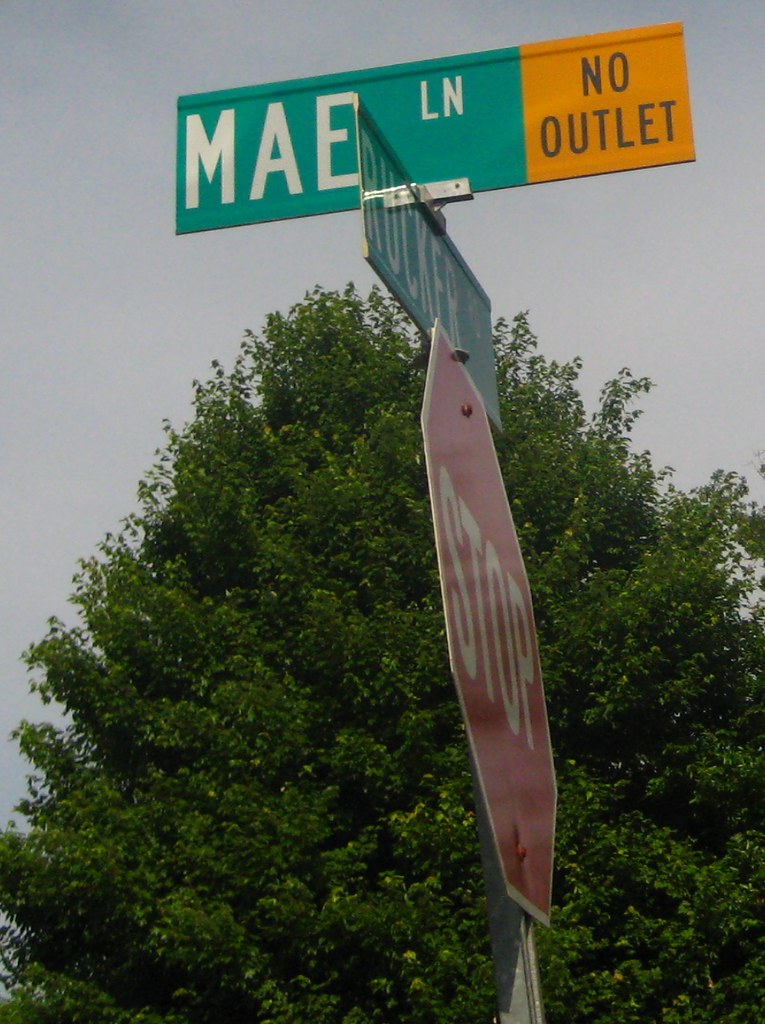The image prominently features a cluster of street signs set against a backdrop of a sprawling tree. The foreground is dominated by a silver post holding a red stop sign, which is angled in such a way that only a partial view is visible. Attached to the same post are two additional signs: one is a green street sign that reads "Rucker Road," and the other is a green and orange sign with the text "May Lane" in the green portion and "No Outlet" in black lettering on the orange portion. The background is filled with a very large tree, its dark green leaves interspersed with occasional patches of light yellowish-green foliage. Overhead, a dull gray overcast sky blankets the scene. The contrasting colors and elements create a visually engaging composition.